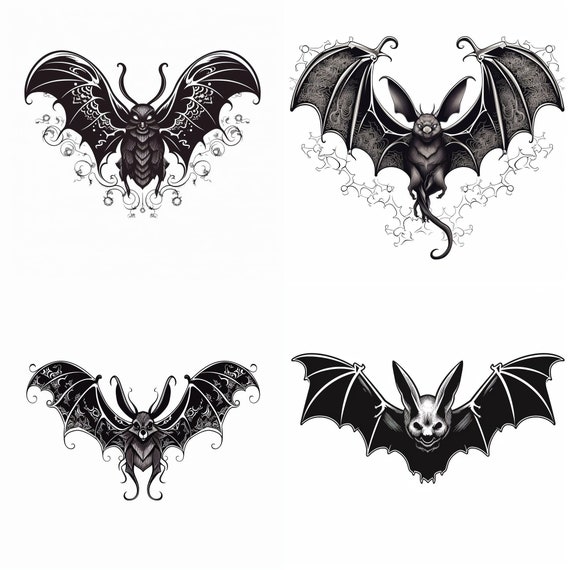The image showcases four intricately drawn bats arranged in a 2x2 grid against a white background. Each bat is depicted in black and white from a frontal perspective.

- **Top Left:** This bat features an insect-like body with long antennae curving outward at the top. Its wings are adorned with wavy patterns and decorative vine-like designs beneath them, giving it an exotic, otherworldly appearance.
  
- **Top Right:** This bat has large, floppy, membrane-like ears and wide wings devoid of any decorative designs. Its wings are a lighter shade, almost gray, and it sports a long, curly tail, enhancing its unusual and whimsical look.

- **Bottom Left:** Resembling a small dog, this bat has a face with black eyes and black wings highlighted with white patterns. The toes of its legs are curled upwards, and unlike the first bat, it is devoid of external flourishes around its body.

- **Bottom Right:** The most traditionally bat-like of the group, this bat has a larger head with long, pointed ears and plain black wings. Its eyes are dark, and the simplistic design underscores its conventional bat features.

The illustrations capture a fascinating variety of bat morphologies, blending elements of fantasy and realism.